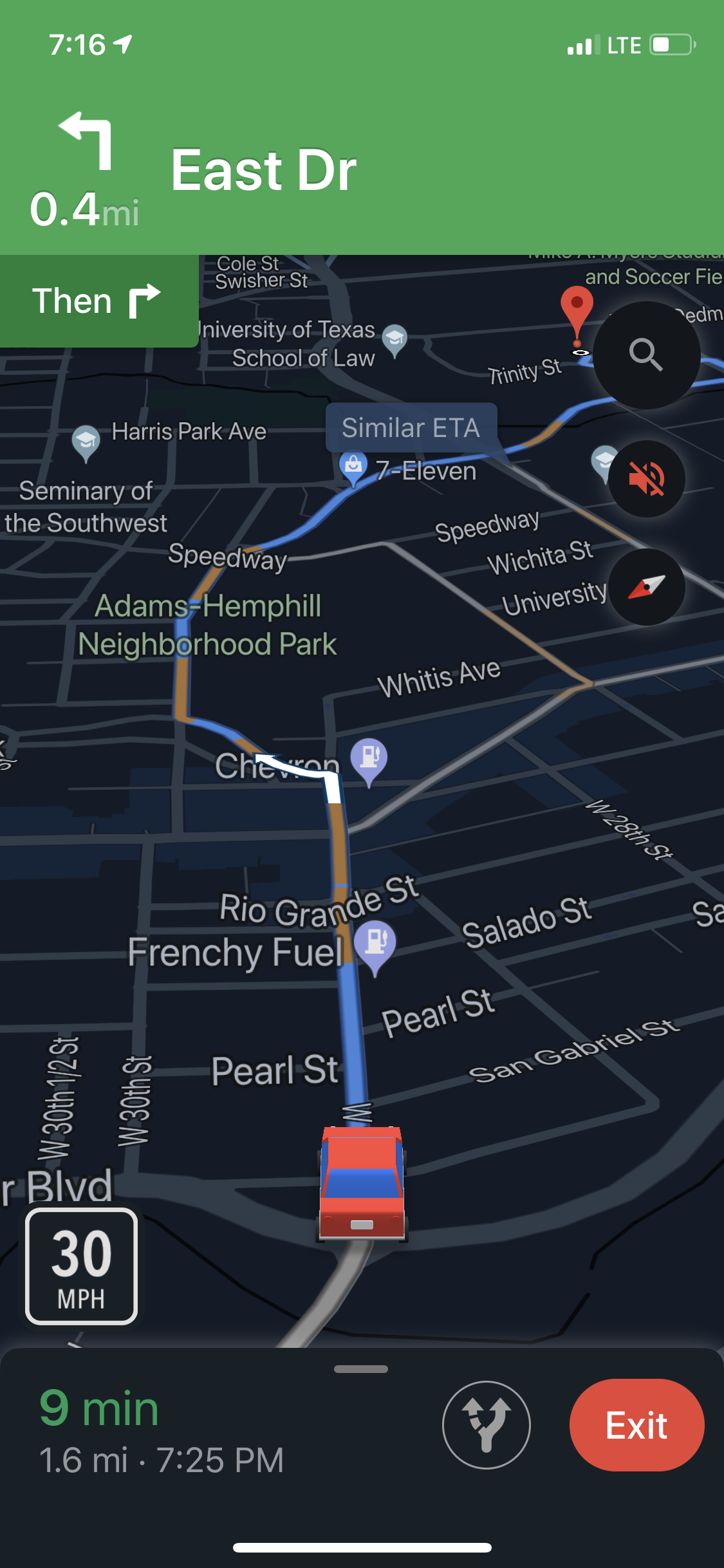A smartphone displaying Google Maps navigation with LTE and a nearly depleted battery (three bars remaining). It is 7:16 PM. The user is searching for East Drive, which is marked 0.4 miles away in green with white text at the top of the screen. Another green bar indicates a right turn ahead. At the bottom left, the speed limit is shown as 30 mph. A 3D red car icon symbolizes the user's current position and navigation route. The bottom of the screen displays an estimated travel time of 9 minutes to cover 1.6 miles. A red exit button is located on the bottom right.

The navigation path requires passing landmarks like Pearl Street, Frenchy Fuels, and Rio Grande Street. The user must turn left at a Chevron, continue by Abram Neff Hills Neighborhood Park, pass a Speedway, and a 7-Eleven. The destination route moves up and to the right, concluding at Trinity Street, just south of a soccer field and east of the University of Texas School of Law. Roads are depicted in light gray, while non-passable blocks are in dark black.